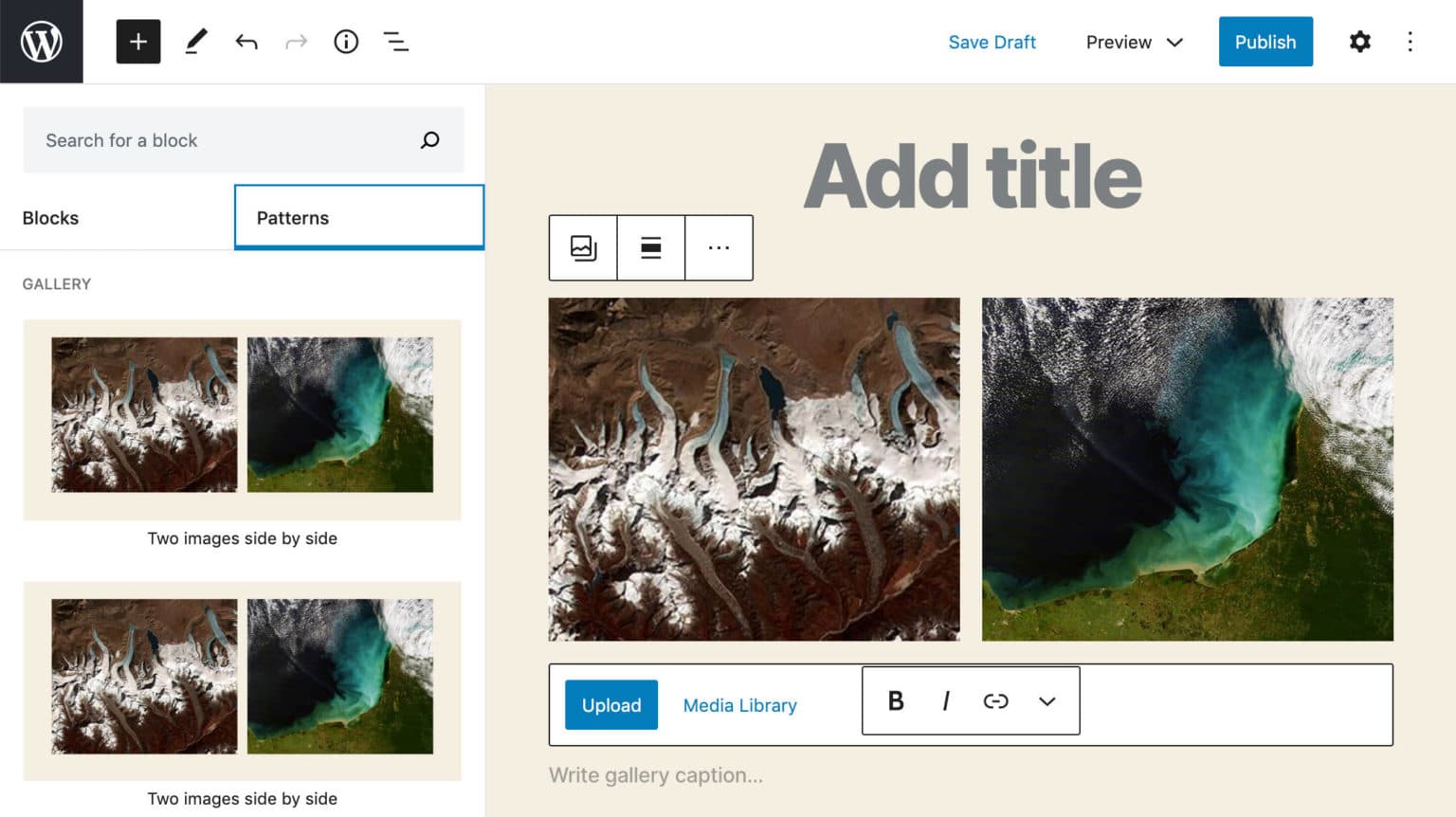The image appears to be a screenshot of a website interface for creating and editing content. On the left, there's a prominent white "W" encircled, indicating a logo, likely representing a web platform or application. Adjacent to it, on the right, is a small black square featuring a white plus symbol at its center, which might be an add or upload button. 

Adding to the interface tools, there is a small pencil logo with an underline, a standard symbol for editing. To the left, there is a black left-pointing arrow and a gray right-pointing arrow, suggesting navigation buttons.

A small "i" encircled, possibly for information or help, is visible alongside three horizontal lines, which likely represent a menu. Further to the right, the words "Save Draft" and "Preview" suggest options for saving and reviewing the content. A notable blue button labeled "Publish" indicates the final step of making the content live. Next to it, three dots signify additional options in a dropdown menu.

The central part of the screenshot displays a picture presumed to be taken inside a cave, adding a visual element to the content. Below the image, there's a distinct blue "Upload" button for adding media, followed by the text "Media Library," providing access to previously uploaded files.

Further down, the phrase "Write Gallery Caption" with an accompanying three dots indicates a section for adding captions to photos in a gallery format. Finally, there's an "Add Title" section, suggesting a space to input the title for the content being created.